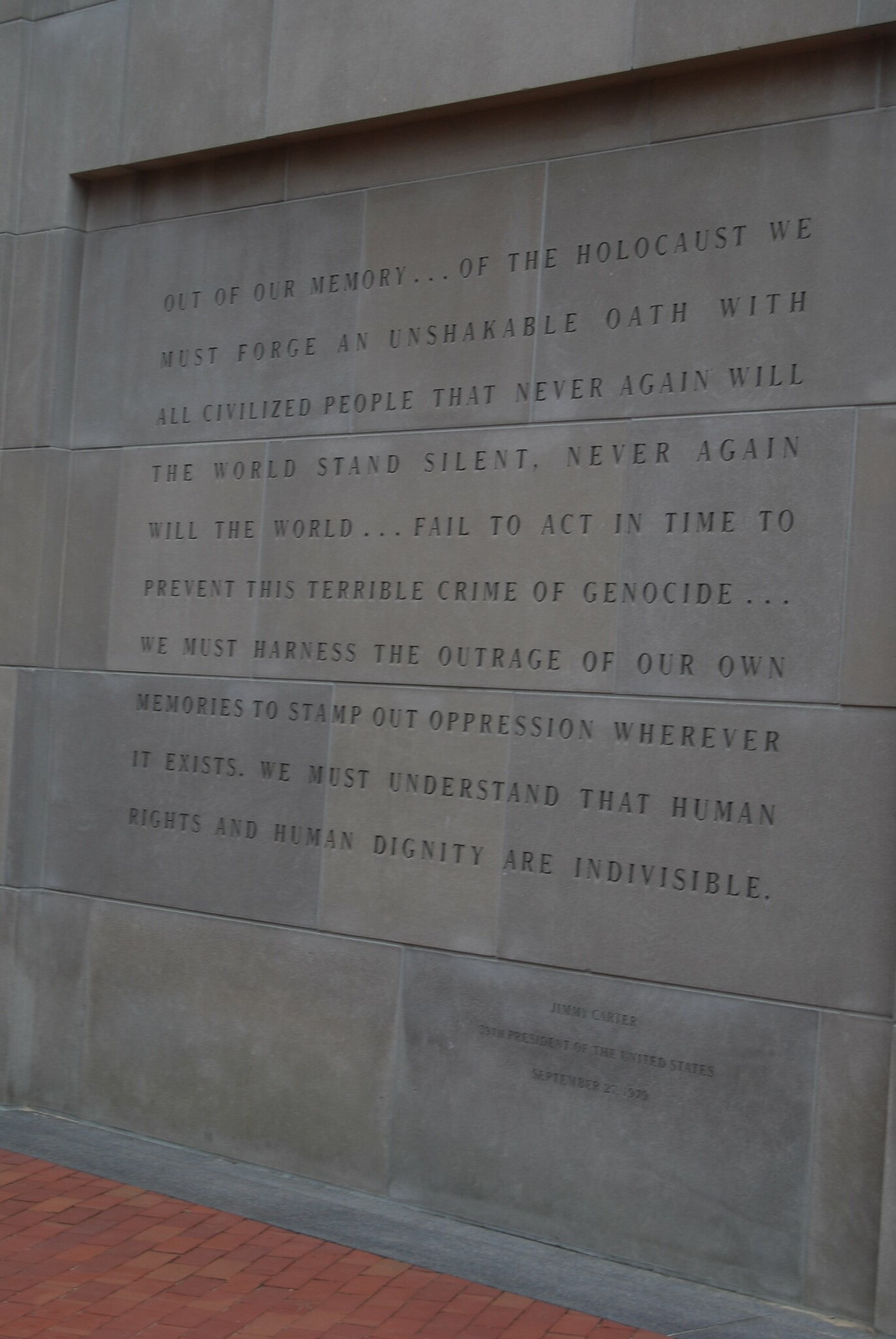This vertically oriented photograph captures an outdoor or indoor space that might be a museum or mausoleum. Dominated by a concrete wall composed of building blocks, it has a section of red bricks on the lower left side. Words are etched into the concrete wall, forming a poignant message about the Holocaust. The inscription reads: "Out of our memory of the Holocaust we must forge an unshakable oath with all civilized people that never again will the world stand silent. Never again will the world fail to act in time to prevent this terrible crime of genocide. We must harness the outrage of our own memories to stamp out oppression wherever it exists. We must understand that human rights and human dignity are indivisible." Despite some difficulty in reading due to the carving, the powerful message is clear and intended to be a lasting reminder for all visitors.